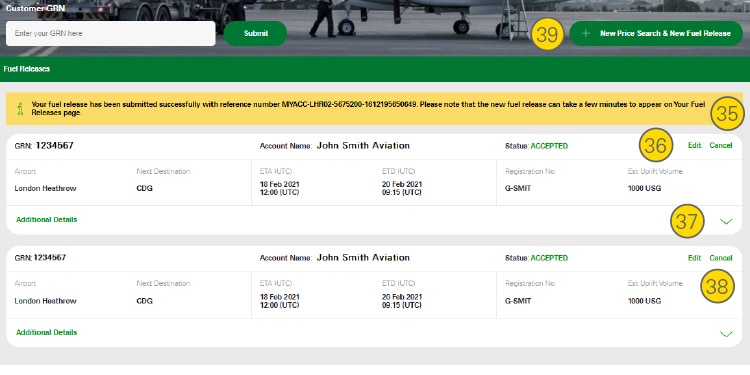This is a detailed and cleaned-up descriptive caption for the provided image:

---

The image is a cropped and edited screenshot from a customer Goods Received Note (GRN) page on an aircraft fueling website. The header section of the page features a black-and-white photograph displaying the wheels of an airplane and a fuel truck positioned on the left side. Superimposed on the image within a text box are the words "Enter your GRN here" in small grey letters, followed by a green oval 'Submit' button to the right. On the far right, there is another green oval button labeled "New Price Search / New Fuel Release," accompanied by a yellow dot with the number "39" in large grey digits, indicating this button's identifier.

Below this header, a green banner with the caption "Fuel Releases" occupies the left side of the screen. Right beneath it, a yellow information banner labeled "35" has appeared, featuring an eye icon on the far left. This alert states, "Your fuel release has been submitted successfully with the reference number: [specific reference number]. Please note that the new fuel release can take a few minutes to appear on your fuel releases page."

Further down, the image displays two listings related to a fuel release for an account named "John Smith Aviation," prominently mentioned at the center top of each box. Each listing indicates its status as "Accepted" shown at the top right corner, followed by 'Edit' and 'Cancel' options marked as "36." A drop-down box for additional details is situated on the far right of each box and designated as "37." At the bottom of these boxes, the registration number and the estimated uplift volume are presented in small grey letters on the right, identified as "38."

---